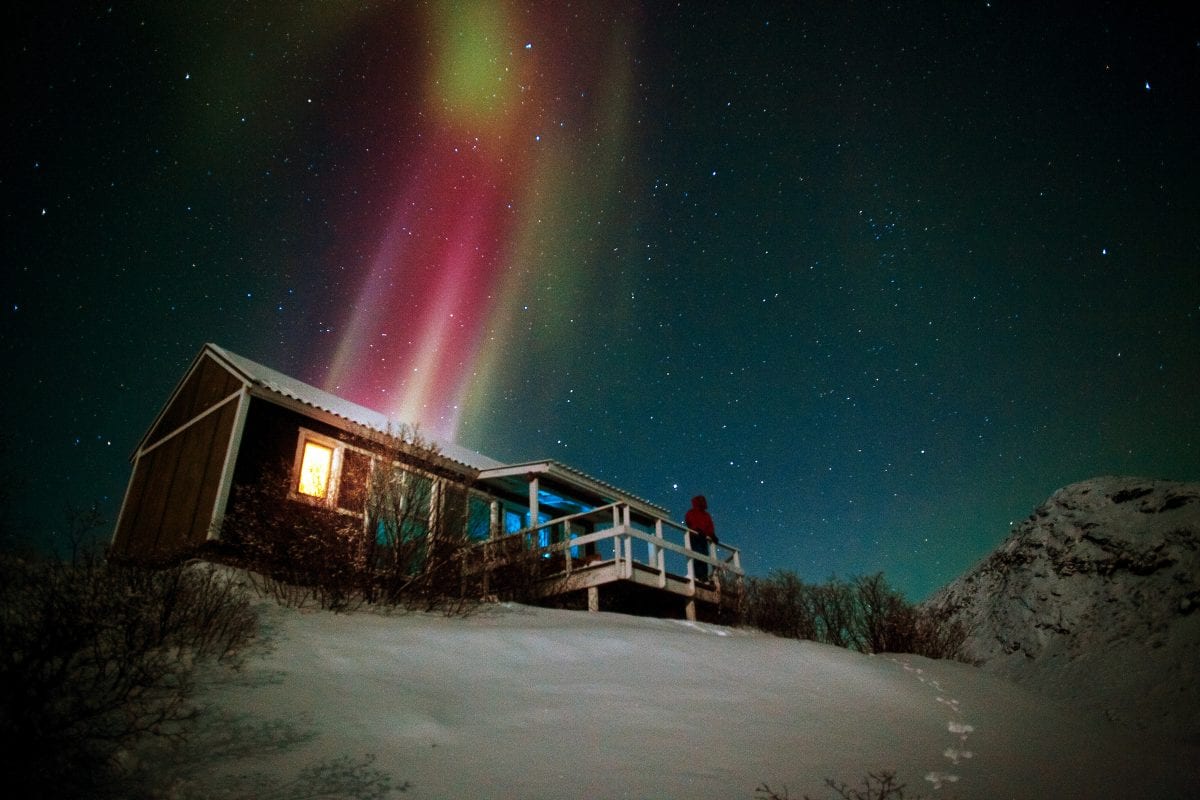In this color photograph taken at night, the stunning northern lights, or aurora borealis, illuminate the sky in a brilliant display of yellow, pink, green, and white. The celestial phenomenon stretches from the top of the heavens down behind a small, one-story cabin with a corrugated roof and a white front porch. The dark, star-filled sky provides a striking backdrop to the colorful streaks of light dancing across it. Below, snow blankets the ground, with a trail of footprints leading up a snowy hill to the cabin. The shrubs surrounding the cabin have bare branches, enhancing the wintery feel. Inside the cabin, a warm yellow light glows from one of the windows, and a faint blue light, possibly from a television, is also visible. Standing on the deck, a person dressed in blue jeans and a long red shirt or hoodie gazes up in awe at the mesmerizing light show in the night sky.